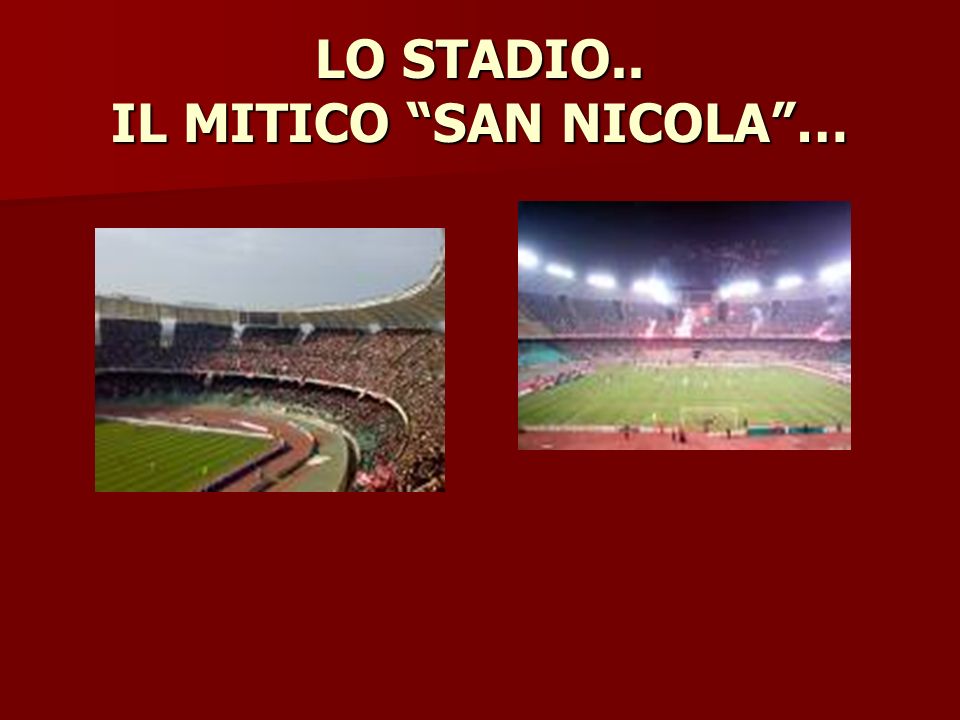In this PowerPoint-style slide, the red background features text at the top written in Italian: "Lo Stadio" followed by "Il Mitico San Nicola." The text is centered and presented in white letters, creating a contrast against the varying shades of red that transition from a lighter hue at the top to a darker, almost maroon shade at the bottom of the slide. Below the text, two slightly skewed images dominate the center of the slide. The image on the left shows a crowded sports stadium with the bright blue sky overhead and a green grass field partially visible, though the picture is cut off at the left and bottom edges. The stands are filled with spectators. The image on the right depicts another stadium under the glow of lights, indicating an evening or night event. In this picture, we see the upper deck of the stands filled with people and a green field, which appears to be viewed from behind a goal. This image is cut off at the right and bottom, and it is positioned slightly higher than the one on the left, adding to the off-centered arrangement of the two images. The scene suggests a lively atmosphere typical of large-scale competitive sports events.